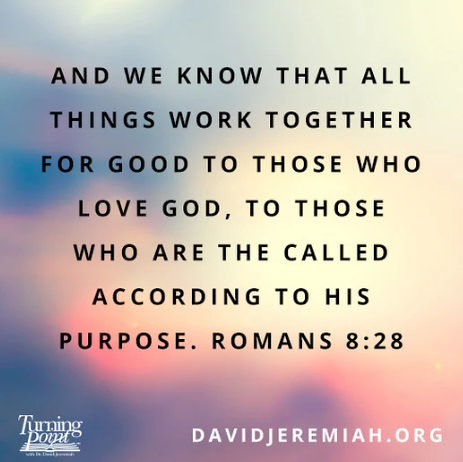The image is a visually striking, inspirational social media post featuring a Bible verse. The background is a colorful, blurred mix of pinks, blues, yellows, and purples, resembling an abstract sunset or a dreamy sky, which helps the text stand out clearly. Centered on the image is a black text quoting Romans 8:28, which states: "And we know that all things work together for good to those who love God, to those who are the called according to His purpose." At the bottom, in white text, the website "DavidJeremiah.org" is noted in the right corner, with the "Turning Point" logo—depicted as a drawing of a book—situated on the left. The image is simple but evocative, designed for easy sharing on social media platforms.